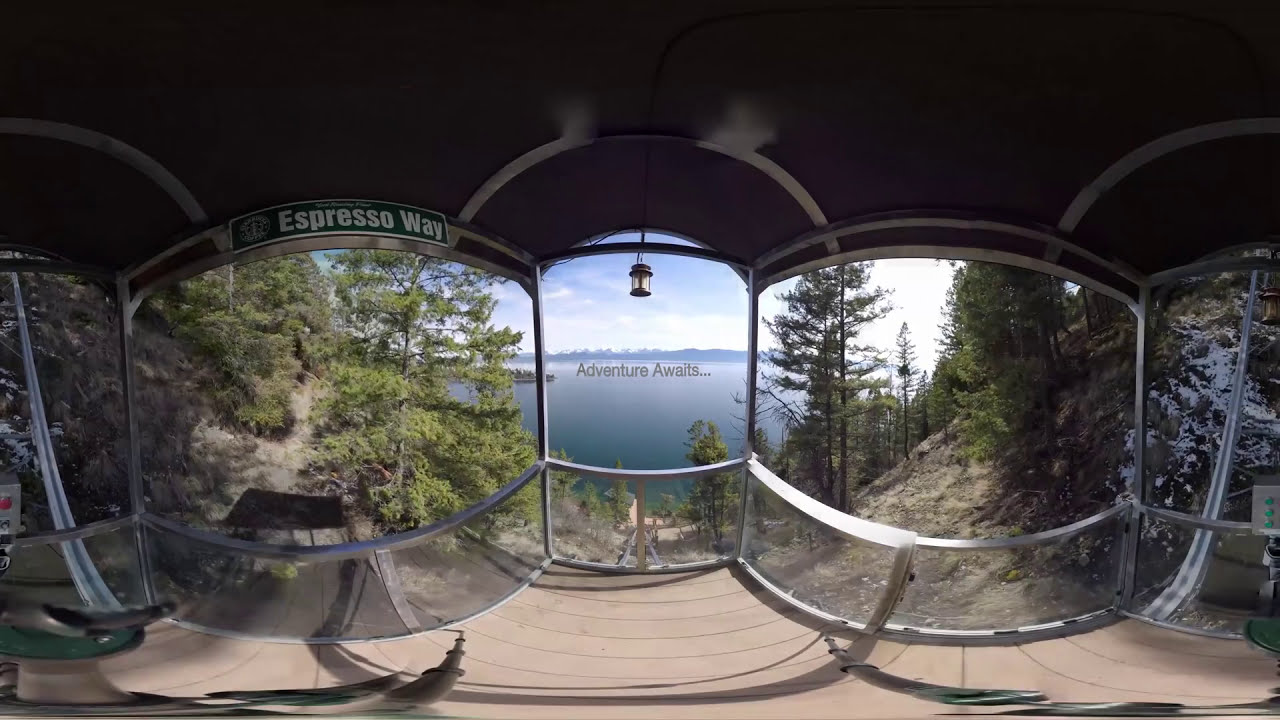This image is a distorted panoramic view taken from a wooden deck or pavilion in a tranquil, forested area. The deck features a black, curved roof supported by archways, and it provides a scenic overlook of a large, calm lake nestled amidst mountains. The lake, expansive in size, mirrors the clarity of the blue sky dotted with clouds. The deck is bordered by a glass and metal railing, and hanging from the center is a small lantern. 

A sign on the left side of the deck reads "Adventure Awaits" in gray text, and another section features a sign that says “Espresso Way” in white font on a green background. The ground leading down to the lake is sloped and populated with numerous trees, some of which have a dusting of snow, suggesting a winter or early spring setting. A control panel is partially visible on the far right side, hinting at some functionality built into the structure. The image was taken during the daytime, with bright, natural light illuminating the scene. The overall composition of the photo suggests that it was taken while moving, causing a warped and curvy appearance to the deck and surrounding landscape.